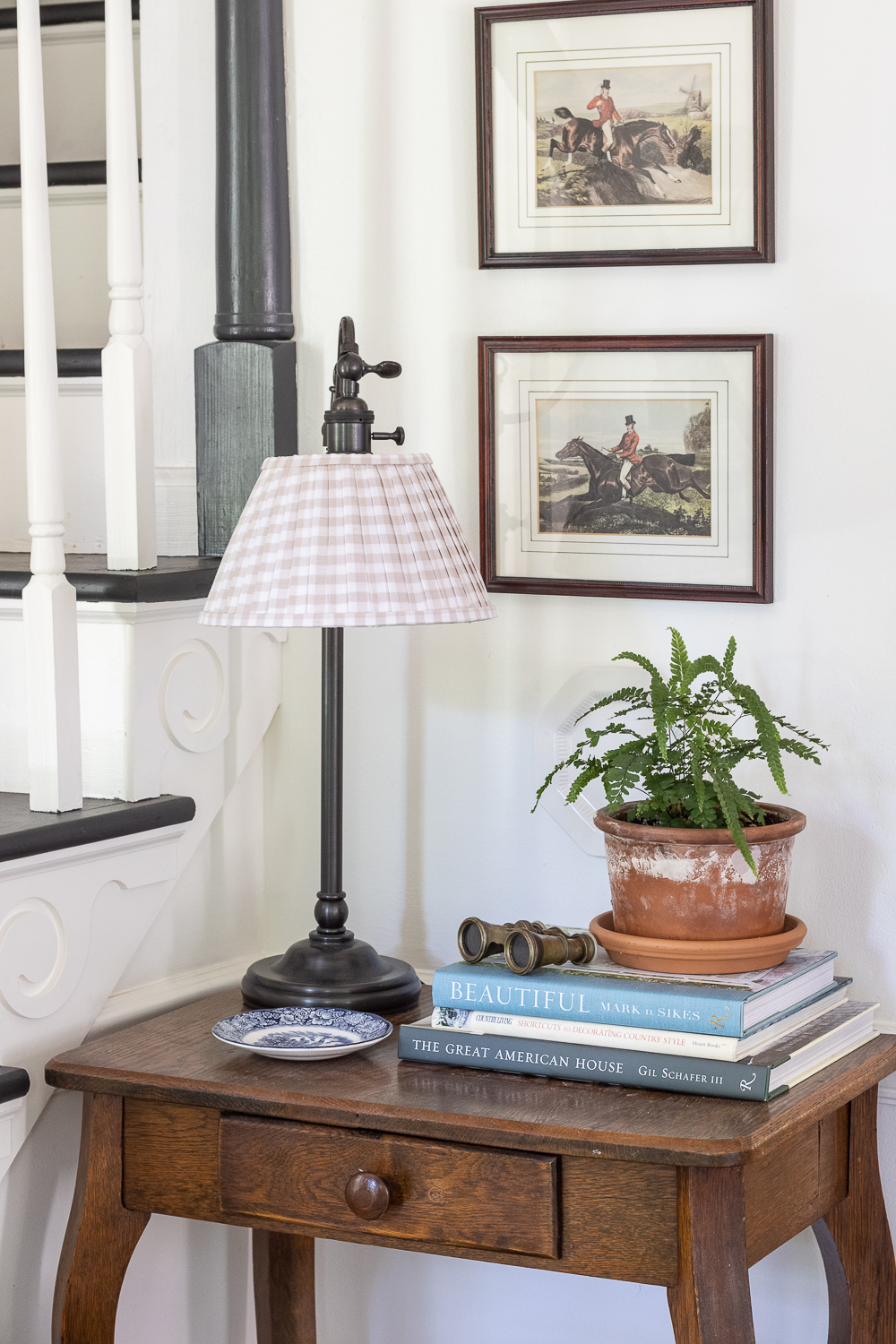In this detailed indoor portrait, a dark wooden desk with a drawer sits adjacent to a staircase featuring black steps and white railings. Positioned against a white wall, the staircase leads the viewer's eye to two framed illustrations of a man on a dark horse. The top illustration depicts the man in red attire and a top hat jumping from left to right, while the bottom one shows him in the same outfit, leaping from right to left. On the desk, an industrial-style lamp with a pink and white shade stands to the left, accompanied by a blue and white ceramic dish. To the right, a stack of books includes titles like "The Great American House by Gil Shaffer III" and "Beautiful by Mark Sykes," with another thin white book in the mix. Atop these books rests a pair of vintage binoculars and a potted plant in a weathered white clay pot on a clay dish. This carefully arranged scene blends vintage decor with a touch of elegance and detail.